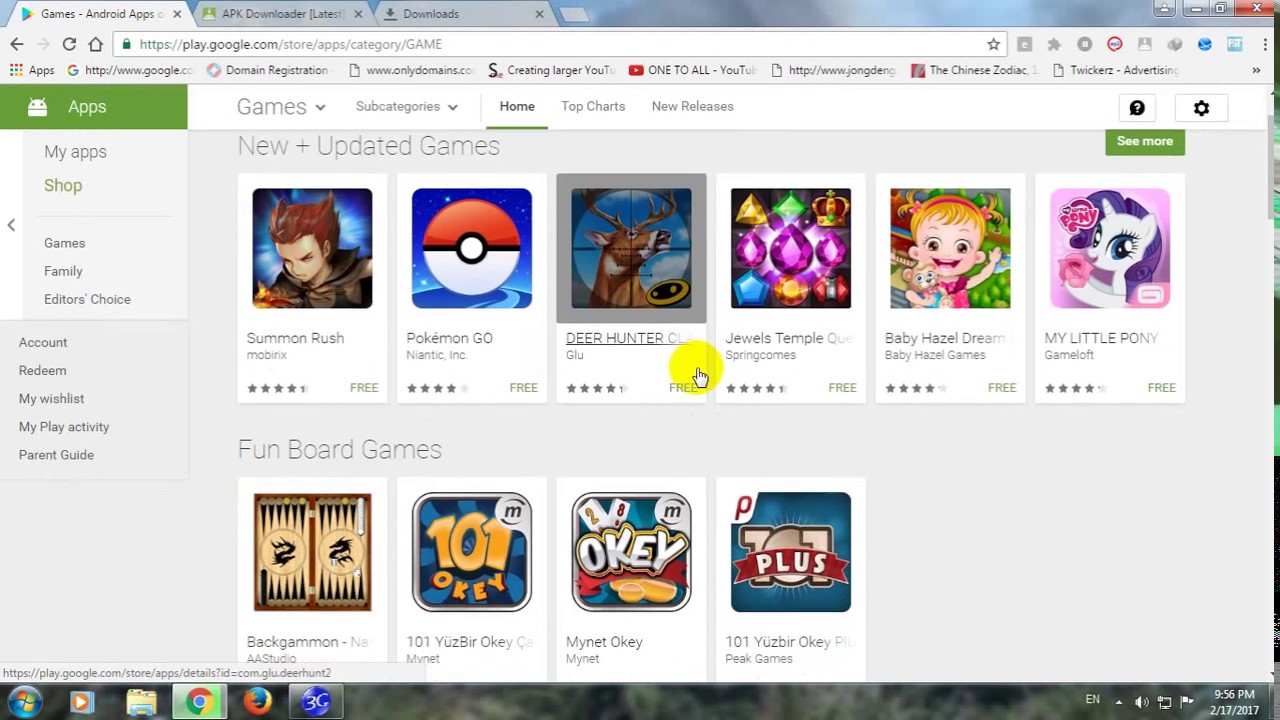A person is browsing the Google Play Store on a desktop computer. In the top left corner of the browser, there is an active tab displaying the Play Store icon and the text "Games – Android Apps." Next to it are two other tabs: one labeled "APK Downloader (Latest)" and another simply titled "Downloads."

The webpage features a navigation sidebar on the left. At the top of this sidebar, there is a green rectangular banner that reads "Apps," accompanied by the older Android mascot, a white alien-like figure. Below this banner, in green text, are the options "My Apps" and "Shop," separated by a gray divider. Further down, in gray text, are the categories "Games," "Families," and "Editor's Choice," all within a light gray background.

The sidebar then transitions into a section with a slightly darker gray background. Here, the options "Account," "Redeem," "My Wishlist," "My Play Activity," and "Parent Guide" are listed.

On the main section of the webpage, the header contains the word "Games" in white, next to a dropdown arrow. Underneath, there is another dropdown for subcategories, followed by a divider. The next option, "Home," is bolded and underlined with a green line, indicating it is currently selected. Other categories listed include "Top Charts" and "New Releases."

Displayed prominently on the page are several game titles, starting with "Summon Rush," followed by "Pokémon Go," "Deer Hunter," "Jewel's Temple," and "Baby Hazel Dream," among others. The subsection "Fun Board Games" features games like "Backgammon," "101 Yüzbir Okey," "My Net Okey," although the text for the latter gets cut off at the end.